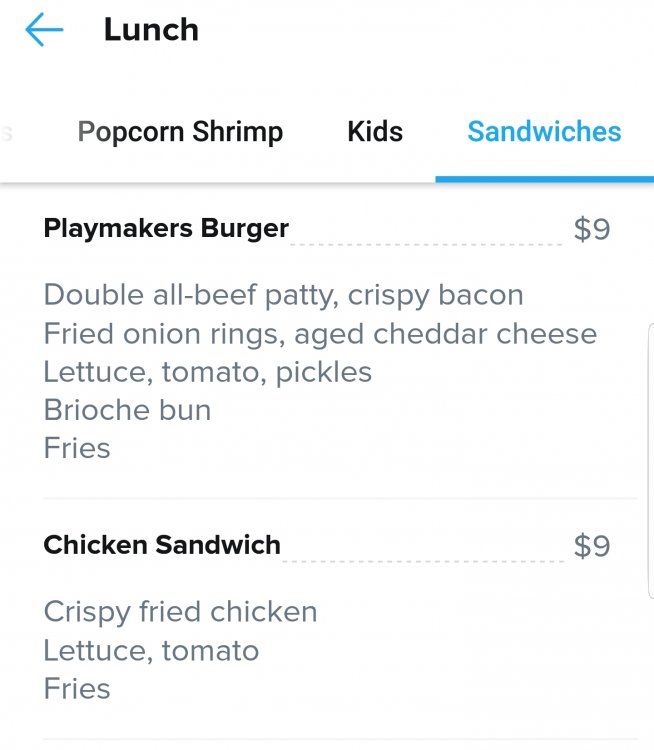The webpage displays a detailed lunch menu featuring various categories such as "Popcorn Shrimp," "Kids," and "Sandwiches." Each category is presented in black text, with the current selection highlighted in blue. The page also includes a back button for easy navigation to the main menu.

Currently focused on the "Sandwiches" section, it lists two options, both priced at $9 and accompanied by fries.

1. **Playmakers Burger** ($9):
   - Double all-beef patty
   - Crispy bacon
   - Fried onion rings
   - Aged cheddar cheese
   - Lettuce
   - Tomato
   - Pickles
   - Brioche bun

2. **Chicken Sandwich** ($9):
   - Crispy fried chicken
   - Lettuce
   - Tomato
  
The Playmakers Burger offers a more elaborate combination of ingredients, including multiple toppings such as aged cheddar cheese and fried onion rings, all served on a brioche bun. In contrast, the Chicken Sandwich is simpler, featuring just lettuce and tomato.

Additional menu categories like "Kids" and "Popcorn Shrimp" are available for those seeking alternatives, although their specific items are not visible in this current view. The restaurant's name is not mentioned on this page.